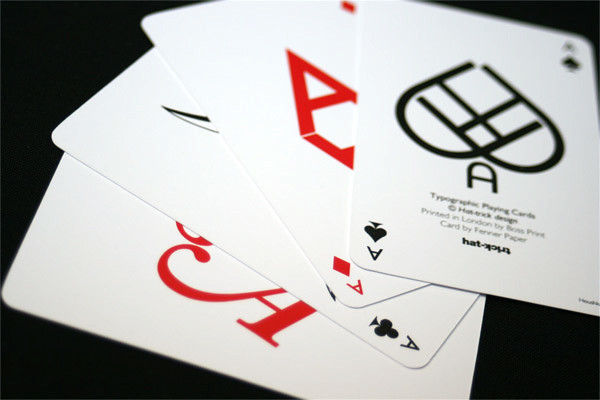This vibrant color photograph captures an extreme close-up view of four playing cards laid out against what appears to be a black tabletop. Prominently featured on the upper right is the Ace of Spades, displaying a large spade icon at its center. Surrounding this icon is some barely readable text, including a blurred company name and the phrase "playing cards," followed by several other indistinguishable lines. Adjacent to the Ace of Spades, on the left, is part of the Ace of Diamonds, identifiable by a red 'A' peeking into the frame. Below and to the bottom right, the corner of another card reveals the identity of the Ace of Clubs. Further left, another partially visible card hints at being the Ace of Hearts, with a portion of the red heart icon discernible in the center. The close proximity and overlapping arrangement of these four aces create a striking focal point set against the contrasting black surface.